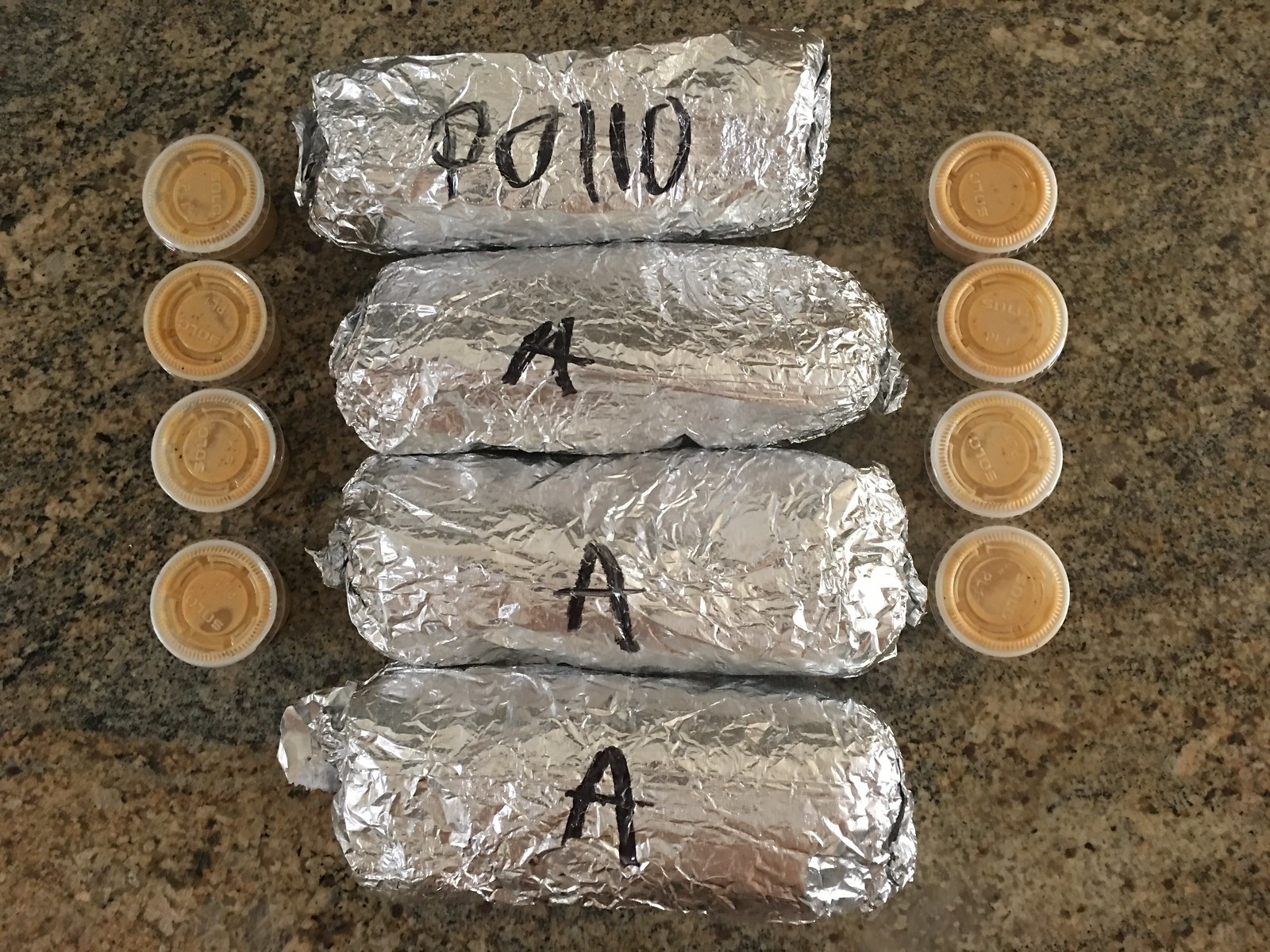A top-down photograph captures a well-lit worktop with a rich, dark brown marble-like surface featuring speckles of tan and black. Centered on the surface are four cylindrical burritos wrapped in shiny aluminum foil, positioned vertically one above the other. The top burrito is labeled "P-O-L-L-O" in black ink, while the remaining three are marked with a capital letter "A" in the same black marker. Flanking the burritos on either side are four small, cylindrical plastic containers with transparent lids, aligned vertically. Each container holds an orange-hued sauce, with subtle reflections of light visible on the foil and the plastic lids, emphasizing the brightness of the setting.